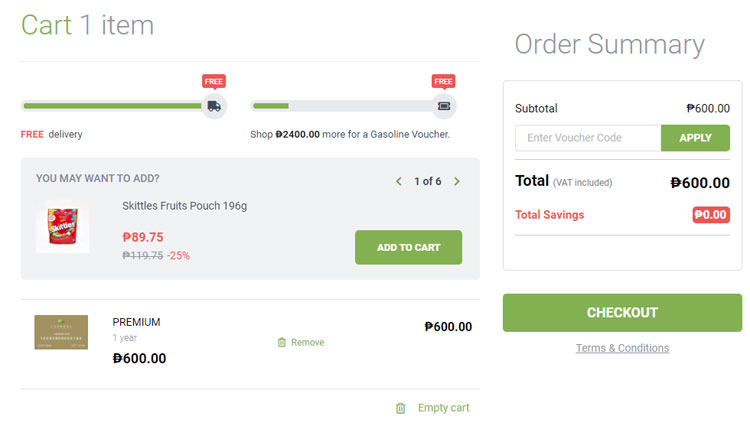The image displays a screenshot of an online shopping cart during the checkout process. The webpage has a clean, white background. In the upper left corner, the word "Cart" is prominently displayed in green, with "1 item" written in gray beneath it. A thin, light line stretches across the width of the page below this.

The image features a progress bar section; the bars are green. The first bar on the left is completely filled, labeled "Free Delivery," while the second bar on the right is about one-eighth filled, labeled "Shop $2,400 more for a gasoline voucher."

Underneath the progress bars, there is a recommendation section with the phrase "You may want to add," showcasing a pack of Skittles Fruit Pouch. To the right of this section is a "Premium" membership offer priced at $600.

On the right side of the image, there is an "Order Summary" box. It shows a subtotal of $600 and a total savings of $0.